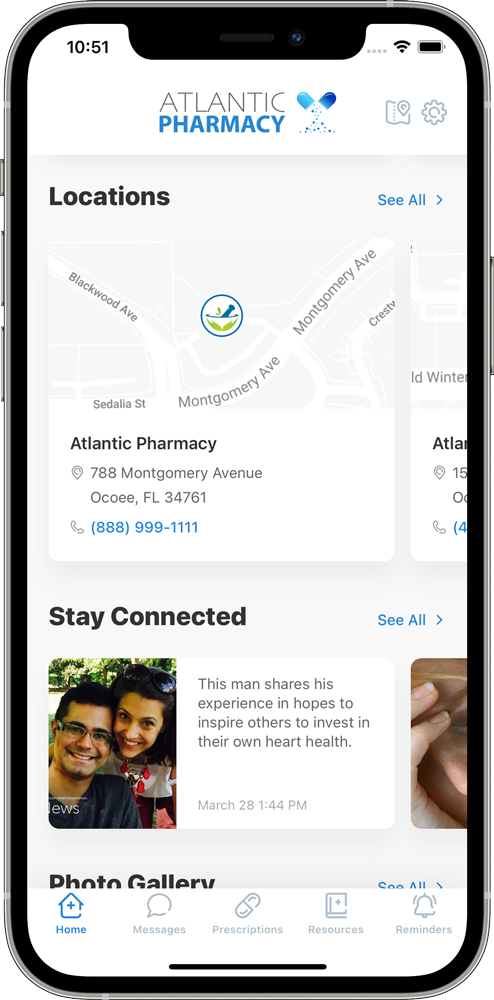Screenshot of the Atlantic Pharmacy Mobile App

In this detailed screenshot of the Atlantic Pharmacy mobile app:

- **Top Bar:** 
  - The time displayed is **10:51 AM**.
  - **Status Icons:** To the far right, there are icons indicating a **Wi-Fi connection** and a **full battery**.

- **Header:**
  - The header shows the title **"Atlantic Pharmacy"**.
    - **Atlantic** is displayed in black, while **Pharmacy** appears in light blue.
  - To the right of the title, there is a capsule pill icon, with two halves pouring out powder, and next to it, there are a small map icon and a coggle (settings) icon, both in gray.

- **Page Sections:**
  - **Locations Section:** 
    - On a slightly gray background, the word **"Locations"** is written in bold black letters. 
    - To the right, there is a **"See All"** link in smaller blue text.
    - Below, there is a map image for **Atlantic Pharmacy**, along with the address: **788 Montgomery Avenue, Ocoee, Florida, 34761**, and a phone number.

  - **Stay Connected Section:** 
    - "Stay Connected" is written in bold black letters.
    - To the right, there is a **"See All"** link in blue letters.
    - This section features a small rectangular story card:
      - The story card shows an image of a smiling man and woman.
      - To the right, on a white background with gray letters, it reads: **"This man shares his experience and hopes to inspire others to invest in their own heart health."**
    - Below this story card, the cutoff of another story is visible, showing only a woman's hand.

  - **Photo Gallery:** The text **"Photo Gallery"** is visible with additional content cut off at the bottom of the image.

- **Bottom Menu:**
  - The bottom menu features icons and labels for **Home, Messages, Prescriptions, Resources,** and **Reminders**, all in gray letters on a white background.

This image offers a comprehensive view of the Atlantic Pharmacy mobile app interface, highlighting the essential navigation elements, contact information, and feature sections designed to keep users informed and engaged.